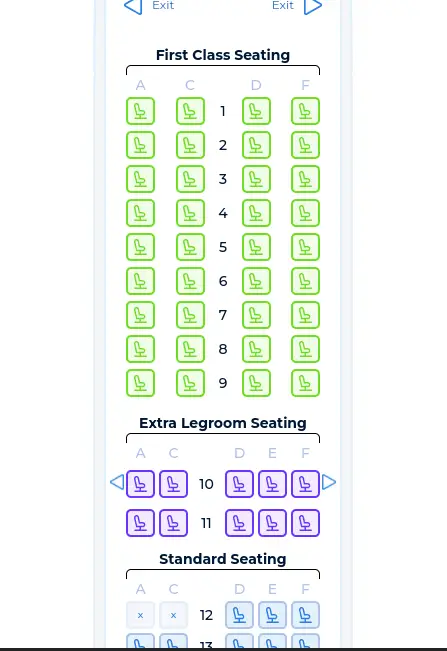A detailed screenshot displaying the seating arrangement options on a flight, likely from a seat selection interface. The section at the top showcases the first-class seating, organized into columns A, C, D, and F. All nine rows in this section are completely available, indicated by green seat icons. Below the first-class section is the extra legroom seating, covering rows 10 and 11. This section includes columns A, C, D, E, and F, with all seats being currently occupied, as marked by purple icons. Further down, the standard seating section is visible, also organized into columns A, C, D, E, and F. The screenshot reveals rows 12 and 13 in this section. In row 12, seats A and C are taken, represented by blue icons with an 'X' over them, while the other seats remain available.